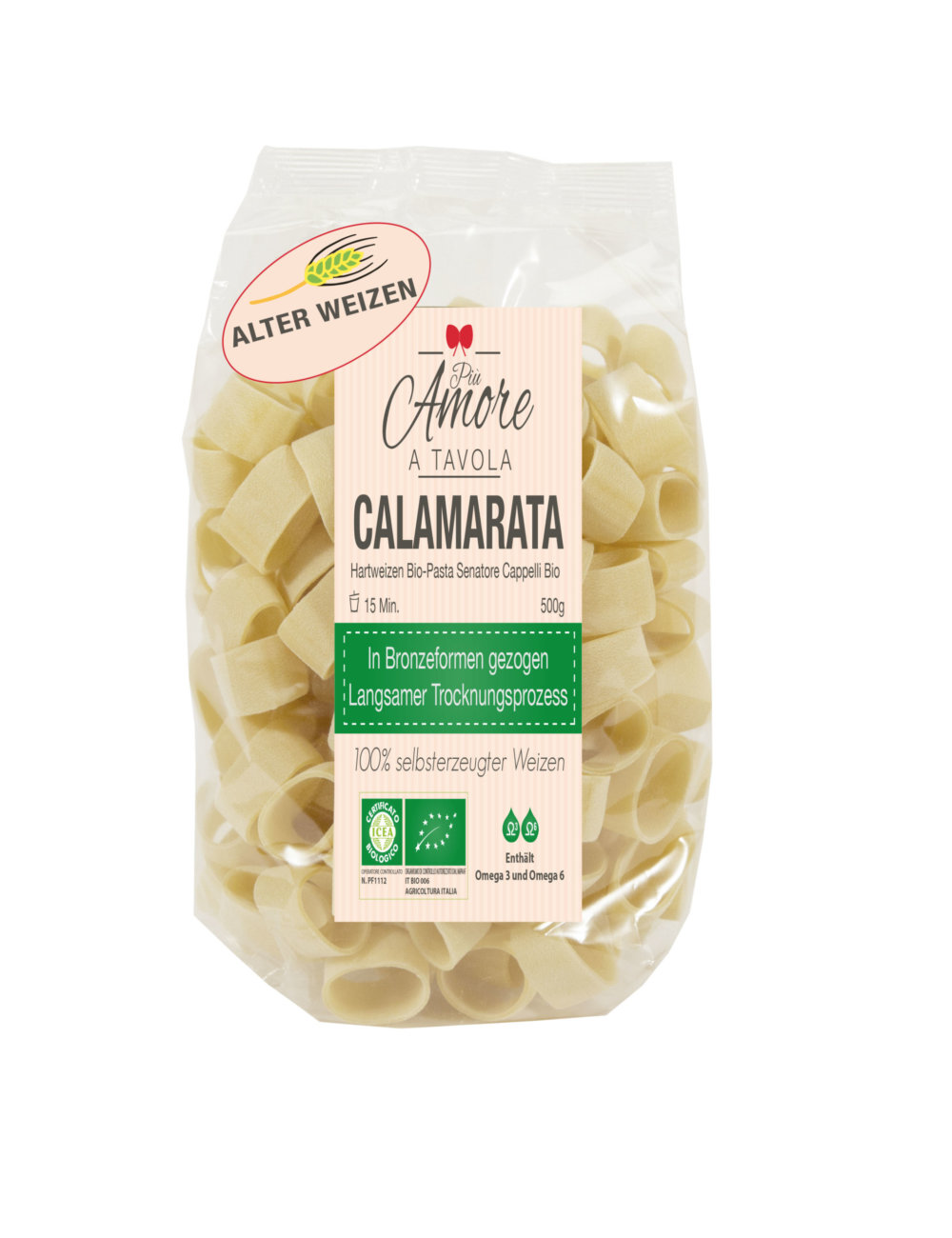The product photo features a single, centrally positioned, transparent plastic packet against a completely white background. The packet contains round, cream-colored noodles and is designed to stand upright, allowing the entire packaging to be clearly visible. The front side of the packet is transparent, providing a clear view of the contents, while the back side is white. A rectangular label is prominently attached in the middle of the packet, featuring text in a foreign language. The label includes various colored fonts in white, off-white, green, yellow, red, and pink. Some of the readable text on the label includes phrases like "Alter Wiesen," "P. Amor A. Tavola," "Cala Marata," "High Sweetsen Bio Pasta Senatore Cappabelli Bio," and the weight "500 grams." The detailed style and positioning of the product suggest that the photo could be intended for use on a supermarket website or in a product catalog.